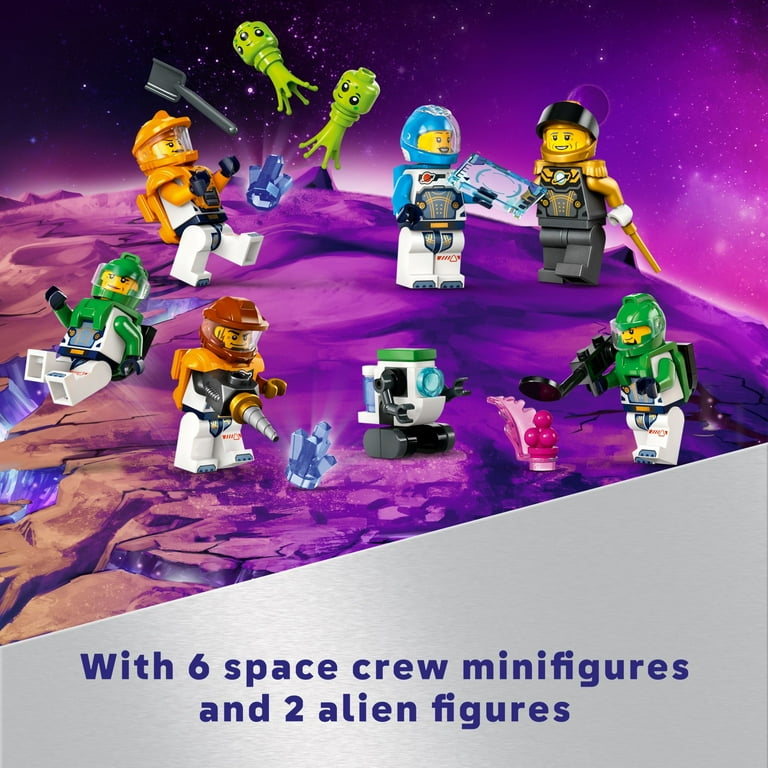The image showcases a vibrant, imaginative scene featuring Lego toys set against a striking purple sky filled with stars and a large purple planet. In the top left-hand corner, there's a black section adding contrast to the scene. Scattered across the image are various Lego minifigures, including six space crew members and two green alien figures. The space crew minifigures are adorned in colorful helmets—orange, blue, green, black, and rust-colored—and outfits in hues of orange, gray, and green. They hold a variety of equipment, such as swords, outer space guns, and other tools, including one with a shovel. The green aliens stand out with their three-eyed heads and peculiar leg-like appendages. The aliens are described as having round bodies with eight feelers. At the bottom of the image, a gray figure and text indicate the presence of "six space crew minifigures and two alien figures." The overall composition suggests an adventurous, space-themed playset against a fantastical cosmic backdrop.